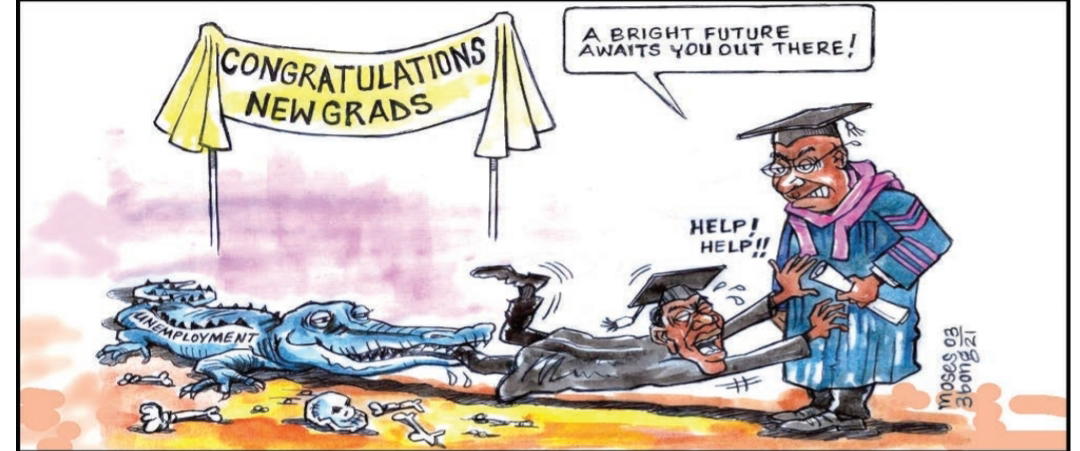In this detailed cartoon image, set against a stark white background, a dramatic scene unfolds featuring a vivid contrast of colors and emotions. On the left side, a bold yellow banner proudly announces "Congratulations New Grads" in black text. The scene is populated by two African-American men, identifiable by their very dark brown skin. One man, dressed in a graduation cap and a blue gown with a pink scarf, is depicted in a state of distress, sweating and exclaiming "Help, help!" as he is being pulled by a blue alligator. The alligator, representing unemployment, has its jaws clamped around the graduate’s leg and appears unconcernedly lazy as it munches away. Nearby, skulls and bones ominously suggest previous victims of this predatory force. The second man, holding a diploma, reassures with a speech bubble that states, "A bright future awaits you out there." Adding to the illustrative composition, the background features accents of yellow and pink, with a purple hue on the left-hand side and the image is signed by the artist Moses 03-3-bong-21 in the upper right corner.